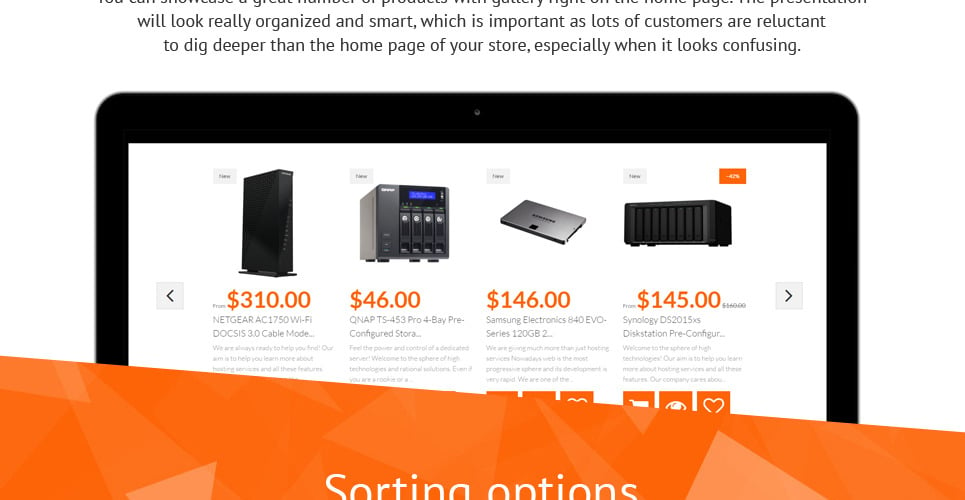**Caption:**

A partial screenshot showcases a tablet with a black casing, displaying a webpage filled with various computer accessories on a white background. The top of the screenshot contains text that reads: "Will look really organized and smart, which is important as lots of customers are reluctant to dig deeper than the homepage of your store, especially when it looks confusing." The tablet screen features a Netgear Wi-Fi cable modem priced at $310, followed by a QNAP TS453 Pro 4-bay pre-configured storage for $46, a Samsung Electronics EVO Series 120GB for $146, and a Synology DS2015XS disk station pre-configuration for $145. All prices are highlighted in orange. At the bottom of the tablet display, a slanted orange banner states "sorting options."